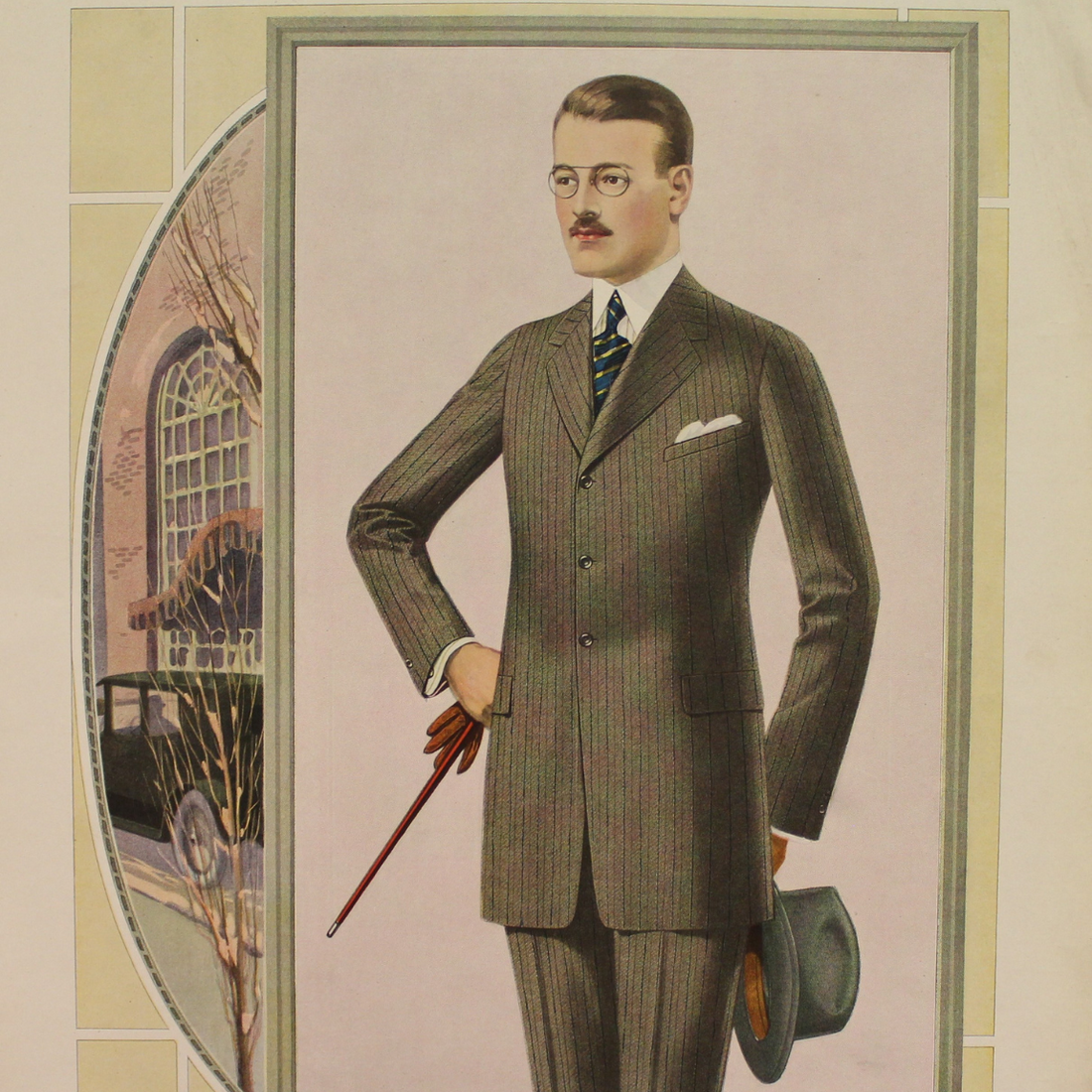The image depicts a detailed, painted artwork of a distinguished gentleman dressed in vintage business attire, reminiscent of the early 20th century. The man is wearing an olive-green pinstripe suit with brown undertones that extends to the middle of his thighs, reflecting the fashion of the 1920s and 1930s. His suit features three buttons and he is accessorized with a white shirt and a blue-and-gold striped tie. The gentleman sports small, circular metal spectacles and has his hair slicked back along with a thin, neat mustache.

In his left hand, he is holding a dark hunter green fedora with a tan interior, while in his right hand, he grasps a brown leather glove and a brown walking stick. To the left of the man, the background reveals a small outdoor scene within an oval frame, depicting a car and a building, hinting that this image might have been sourced from an older book.